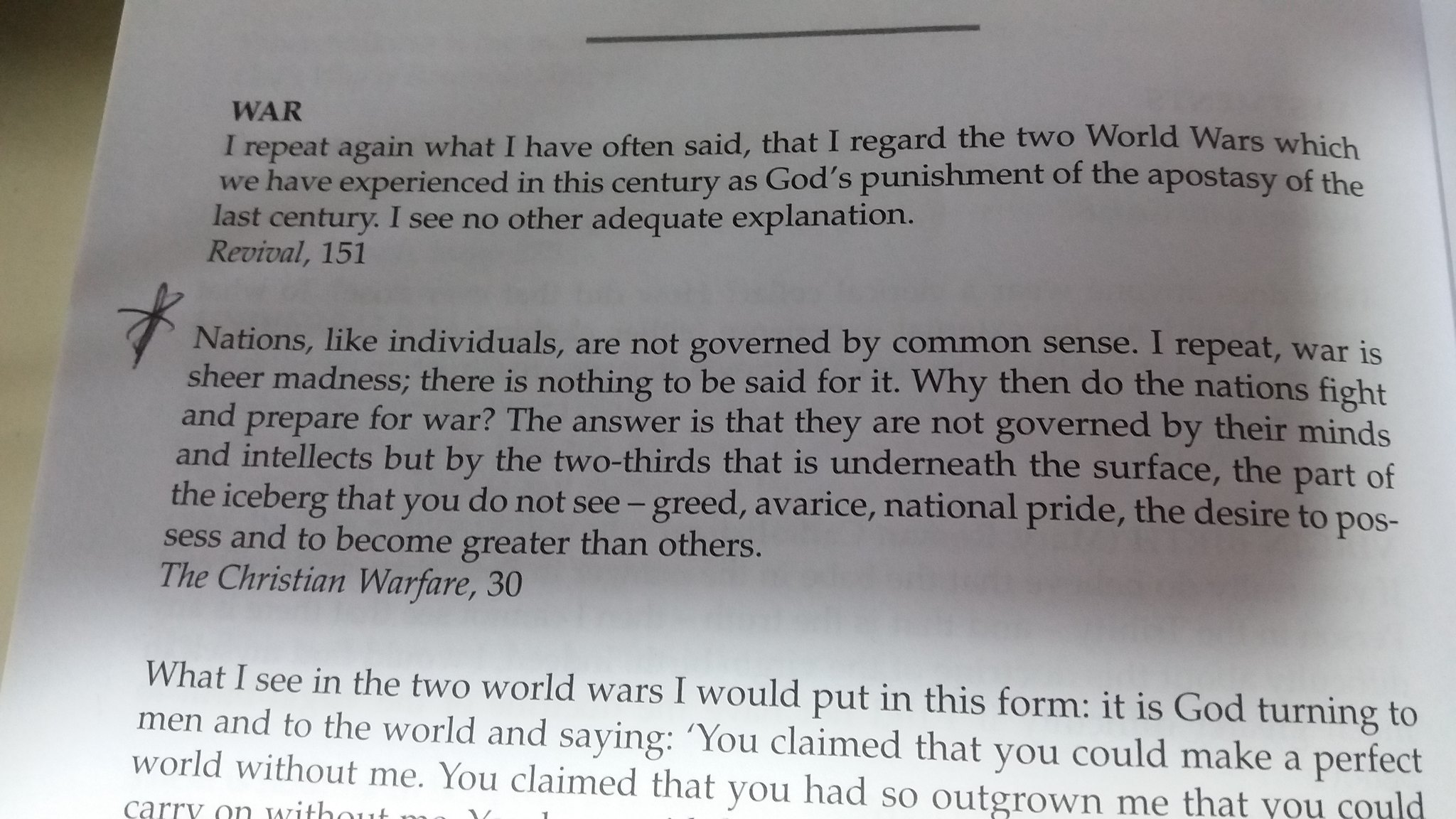The black-and-white image depicts a page from a book with black print against a white background. At the top, in bold letters, is the title "War." Below the title, the text discusses the two world wars as divine punishment and includes a citation to "Revival, 151." A notable detail is a handwritten asterisk in the margin next to a paragraph emphasizing that nations, like individuals, are driven by hidden motivations like greed and pride, rather than common sense. This starred section, part of which reads "Nations like individuals are not governed by common sense. I repeat, war is sheer madness," is a quote from "The Christian Warfare, 30." The image displays a stark contrast in lighting: the top part of the page is shadowed, while the bottom part, where the last paragraph resides, is brightly lit, possibly due to light hitting that area.